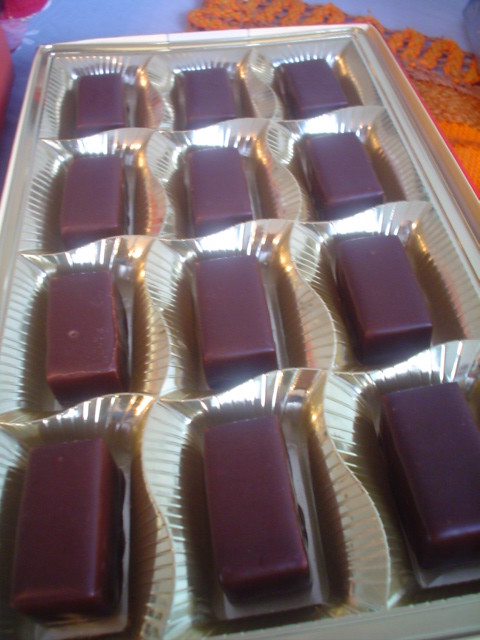The image depicts an intricately molded golden plastic tray holding 12 rectangular chocolate candies. Each chocolate is about an inch tall and covered in a dark, reddish-brown chocolate. The molded tray, designed with curved ruffled lines reminiscent of seashells, contains individual nooks for each piece of candy, ensuring they remain separated and intact. This tray, placed on a blue table, is lined with a white material to prevent sticking. Behind the tray, a bright orange placemat with tassels on its ends lays flat, adding a vibrant backdrop. To the top left corner of the tray, there are two pieces of red fruit, likely apples, adding a contrasting color to the arrangement.